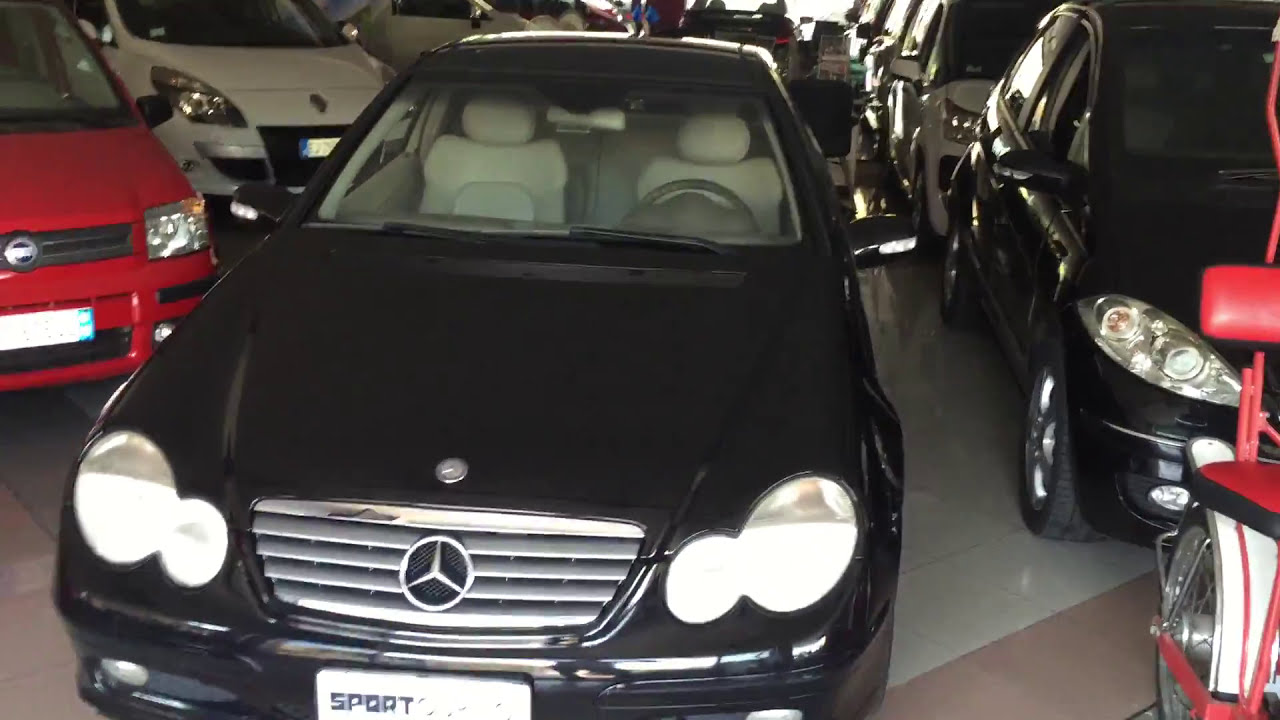In this horizontally aligned rectangular image, we are viewing the front of a sleek black Mercedes-Benz, prominently displayed indoors on a white and brown tiled showroom floor. The vehicle's front grille features a gray and chrome finish, complete with the iconic Mercedes-Benz logo prominently on the hood and bumper. A partially visible license plate reads "Sport," though the plate is cut off at the bottom of the picture. The car boasts gray leather seats and a black steering wheel inside.

Surrounding the Mercedes-Benz, the showroom is packed with various other cars. On its left, a red car is parked at an angle, with a white car positioned behind it. To the right, directly aligned with the black Mercedes, is another black car, followed by a white car behind it. Interestingly, on the far right, there appears to be a motorized vehicle, possibly a scooter or bike. The showroom floor is shiny, resembling marble, adding to the luxurious atmosphere. In the background, a desk and a window can be faintly seen, with light streaming through and possibly a person seated at the desk, though the details are a bit blurry.